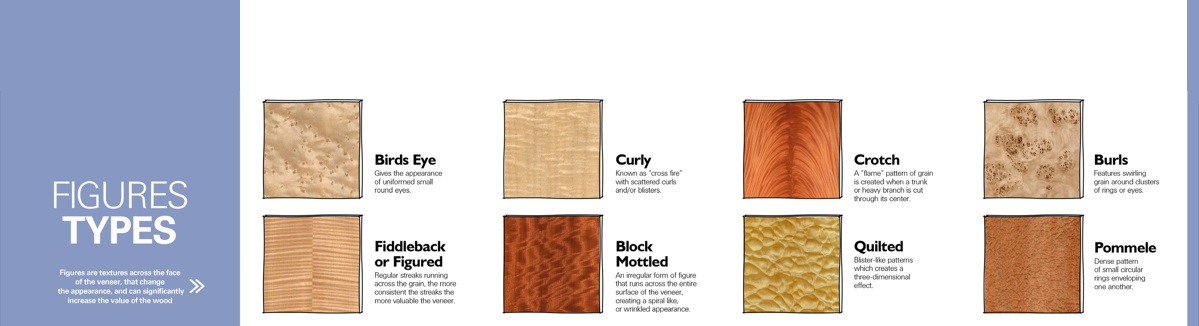The image is a detailed poster titled "Figure Types" displayed in a blue rectangular box on the left side. The poster showcases eight different wood patterns arranged in two rows of four columns each. The samples, varying in shades of brown and yellow, are labeled as follows from left to right and top to bottom: 

1. Bird's Eye - Exhibits a uniform, sandy-colored appearance with small, round eyes.
2. Curly - Known as crossfire, it features scattered curls.
3. Crotch - Displays a flame pattern created when a trunk or heavy branch is cut through its corner.
4. Burls - Shows an uneven grain pattern.
5. Fiddleback or Figured - Characterized by regular streaks running across the grain, the more consistent the streaks, the more valuable the veneer.
6. Block Malted - Exhibits a distorted texture.
7. Quilted - Appears bumpy.
8. Pommel - Features dense patterns of small circular rings enveloping one another.

Each wood figure type has a description underneath its name, though the text is too small to be clearly legible. The visual detail in the samples highlights the unique textures and patterns found in different types of wood.